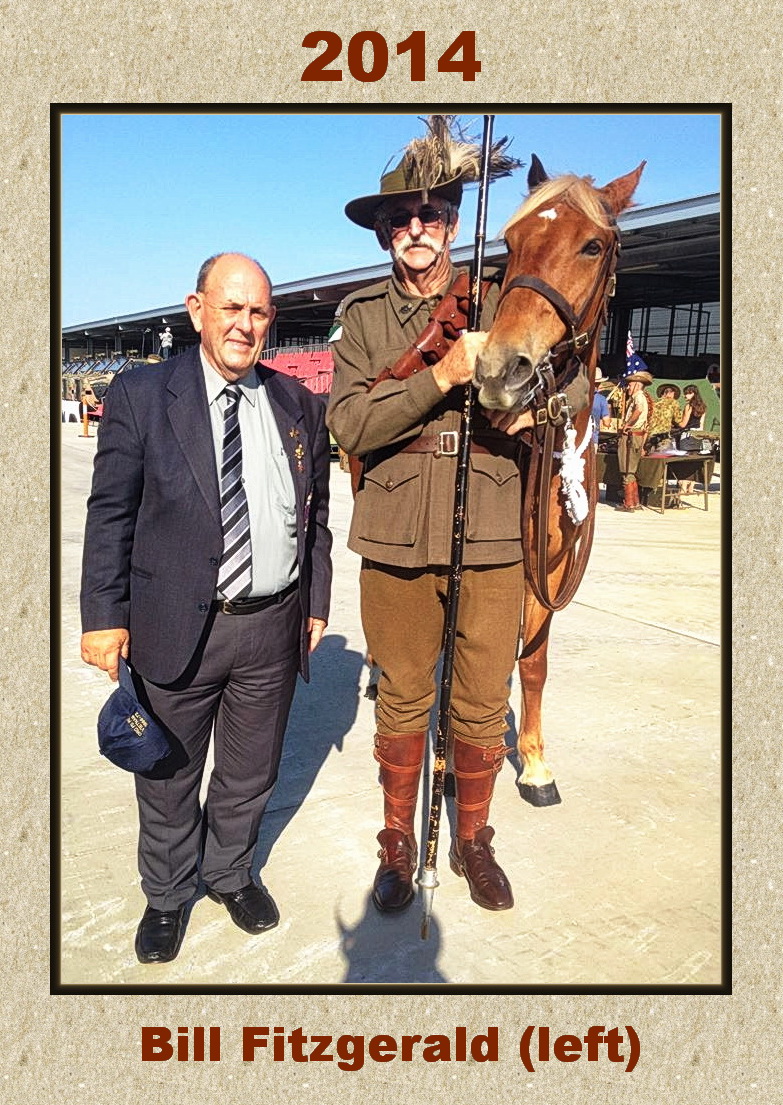In this photograph taken outside on a clear blue day, two men stand side by side with a horse. On the left is a short, balding man dressed in a dark suit with a white collared shirt and a black-and-silver striped tie. He holds a blue baseball cap in his hand, squinting slightly in the sunlight. To his right is a taller man in a vintage military outfit, primarily shades of brown, including a brown safari jacket, pants, boots, and a distinctive hat with feathers. He sports sunglasses and a white handlebar mustache, giving him a striking appearance. Leaning over his left shoulder is a tall brown horse with a blonde mane and a white mark on its head. The horse's body is partially obscured, with one leg visible. They are standing on a sandy surface in front of a large metal building with tables set up in front. The image is framed by a textured brown border with "2014" inscribed at the top and "Bill Fitzgerald left" at the bottom.